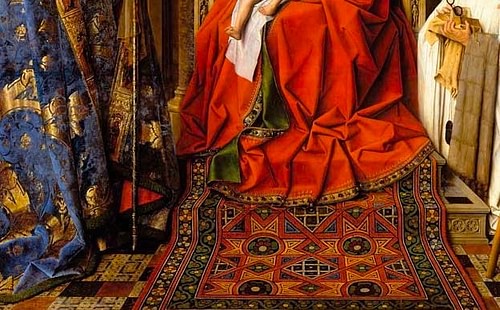This is a close-up section of a heavily cropped painting, presenting a rich tapestry of colors and textures. The central figure appears to be an adult seated on a throne, draped in an elaborate red robe adorned with golden designs and accented with touches of green. The individual's large robe partly obscures a glimpse of small children's feet resting in their lap, wrapped in a white sheet or blanket. Below the throne, a detailed throw rug with a diverse pattern of geometric shapes and vibrant colors such as yellow, blue, red, and orange covers the steps. To the left, part of another figure is visible, clad in a similarly ornate blue garment with gold designs. This figure might be holding a staff or sword, lending to the impression that they, too, are part of a regal or formal scene. The painting, though lacking its upper half, suggests a narrative of grandeur and intimacy set against a backdrop of intricate fabrics and meticulous craftsmanship.